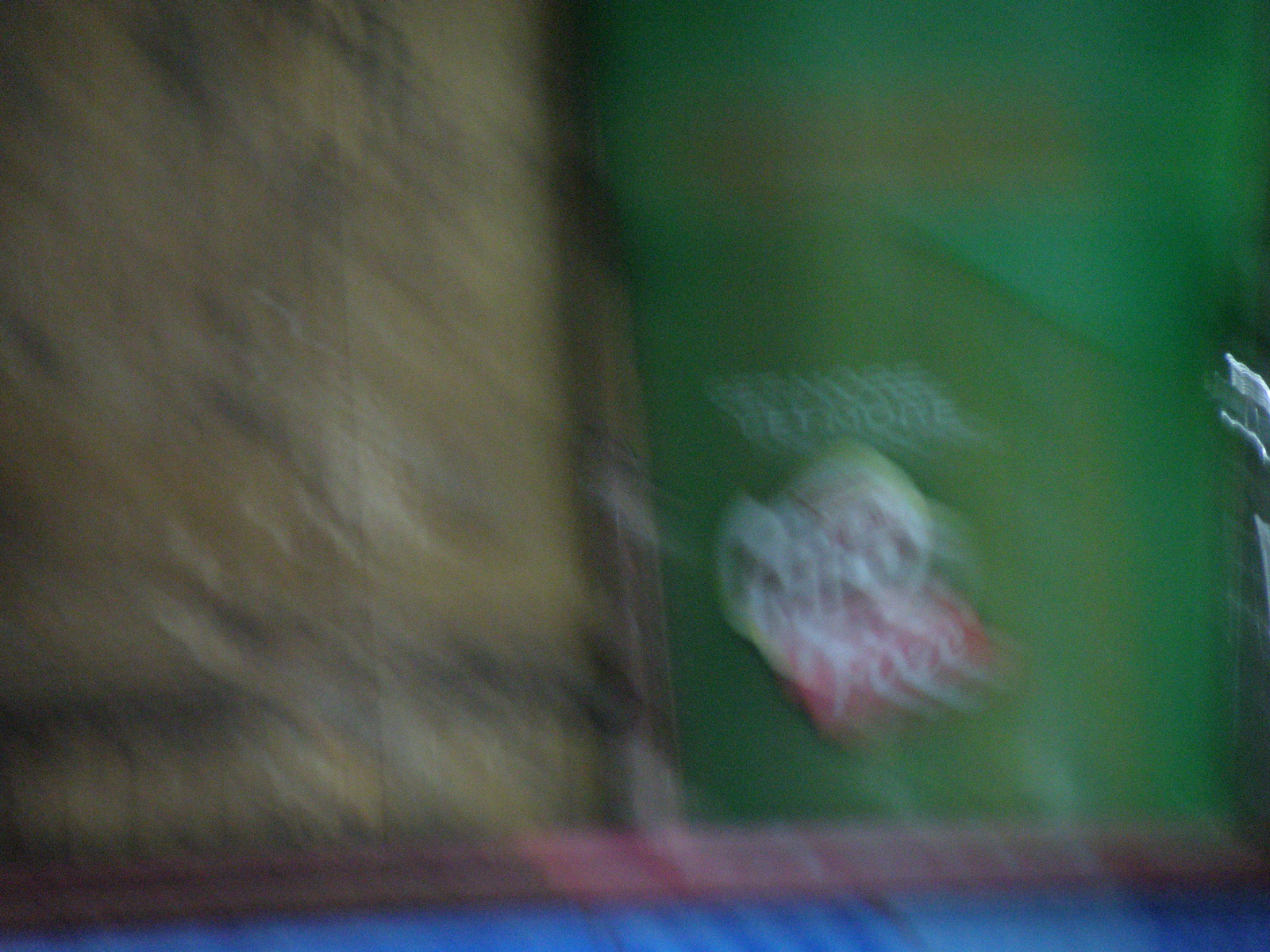The image depicts a blurred photograph likely taken with a shaky camera, giving the impression of motion. Dominating the left side of the image, there is a green container with the white text “GET MORE” clearly visible. Next to it is a symbol or logo, possibly saying "MILO" or "MIDO", accompanied by additional red and white text, though it’s hard to decipher. On the right, there is another container, this one brown, with hints of black, positioned on what appears to be a brown shelf. The bottom of the image is tinged with blue, suggesting the presence of a blue surface or lighting below. The photo, seemingly taken in a dimly-lit environment with natural light, features six distinct colors: red, white, brown, green, black, and blue, creating a vibrant but unclear scene possibly set in a store, restaurant, or pantry storage area.